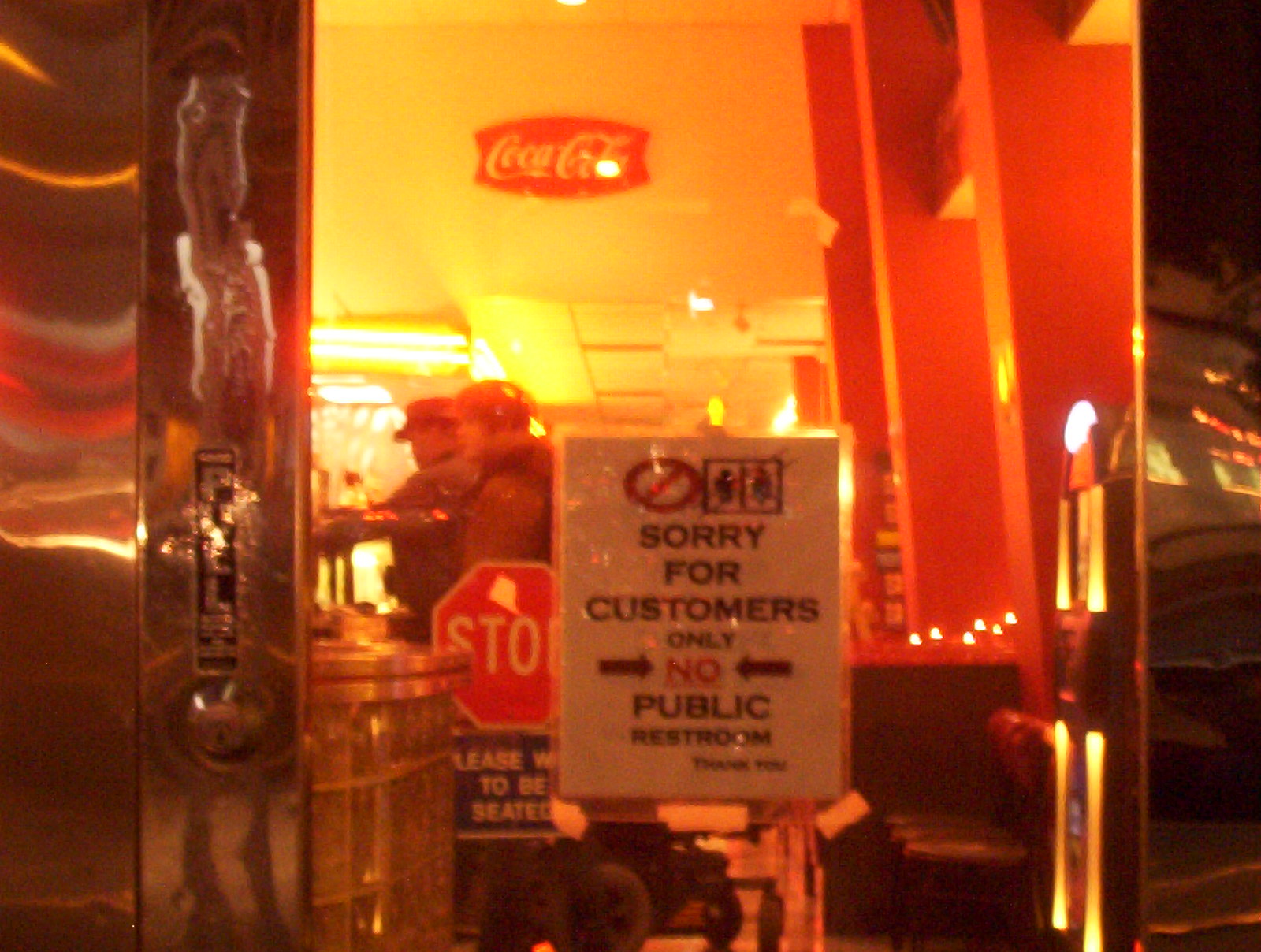The image appears to be taken through a glass door with a stainless steel frame, capturing the inside view of a restaurant or diner. The glass door prominently displays a white rectangular sign that reads "Sorry, for customers only. No public restroom." Upon closer inspection, the perspective seems to add a yellow and orange hue to the scene, possibly as if the photo was taken through a tinted or translucent object. The framing at the top features a Coca-Cola sign, lending a nostalgic touch. Inside the diner, to the right, there is a jukebox and several people can be seen. A significant detail is the stop sign accompanied by a "Please wait to be seated" notice, situated a bit further into the restaurant. The walls are painted orange and the lighting has a warm, yellow glow, contributing to the cozy and inviting ambience of the diner.